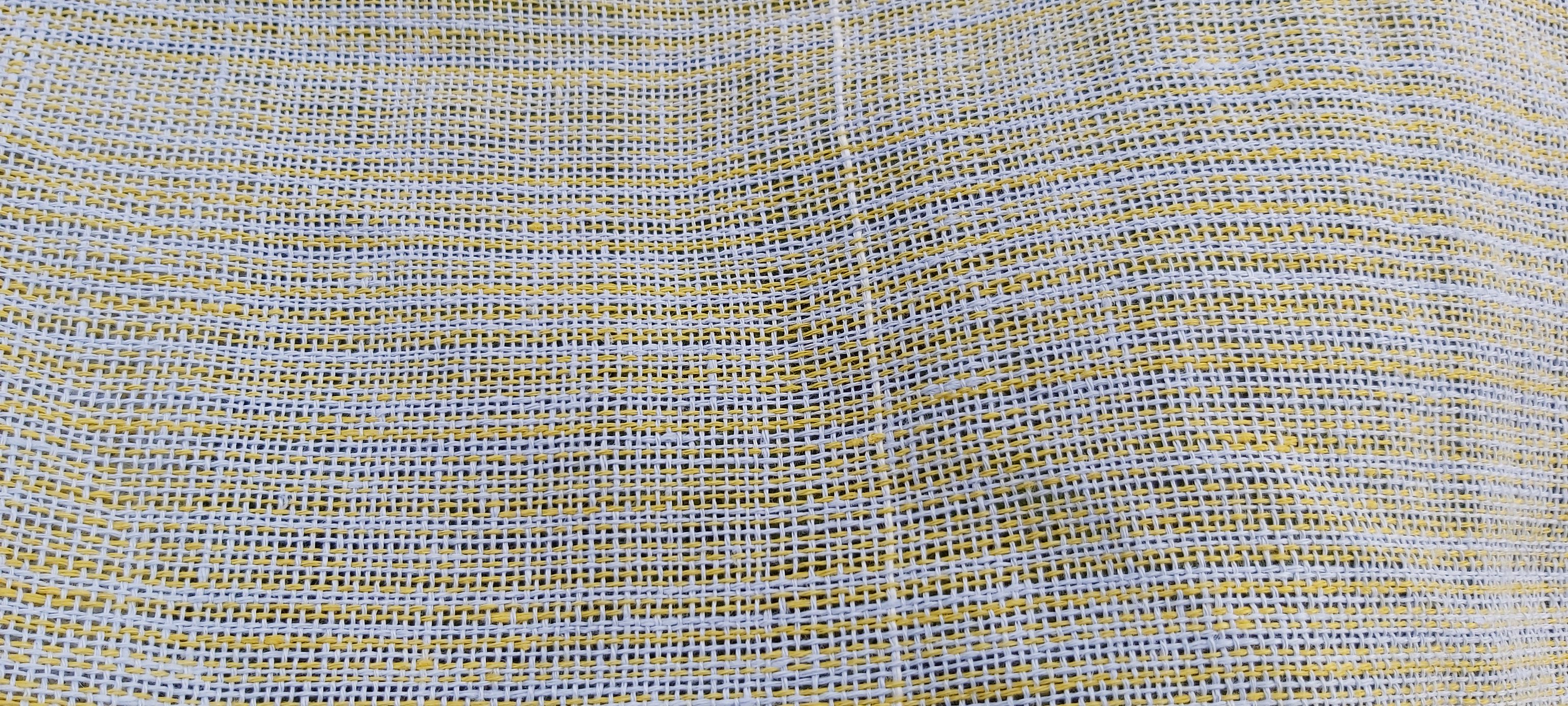This close-up image features an intricately woven piece of fabric with a loose weave, allowing clear visibility of the gaps between the threads. The fabric exhibits alternating stripes of yellow and white that vary in thickness, sometimes showing consecutive streaks of the same color, creating a pattern that resembles thick blended lines. The cloth's texture suggests a screen door effect, emphasizing its transparency. There is a slight curve towards the right-hand side of the fabric, indicating it's not completely flat. A notable element is a thicker, darker vertical white thread running through the center, which stands out against the horizontal weave, potentially signifying a seam or a variance in thread thickness. The material evokes a feeling similar to cheesecloth and could be used for items like tablecloths or coverings that require breathability.